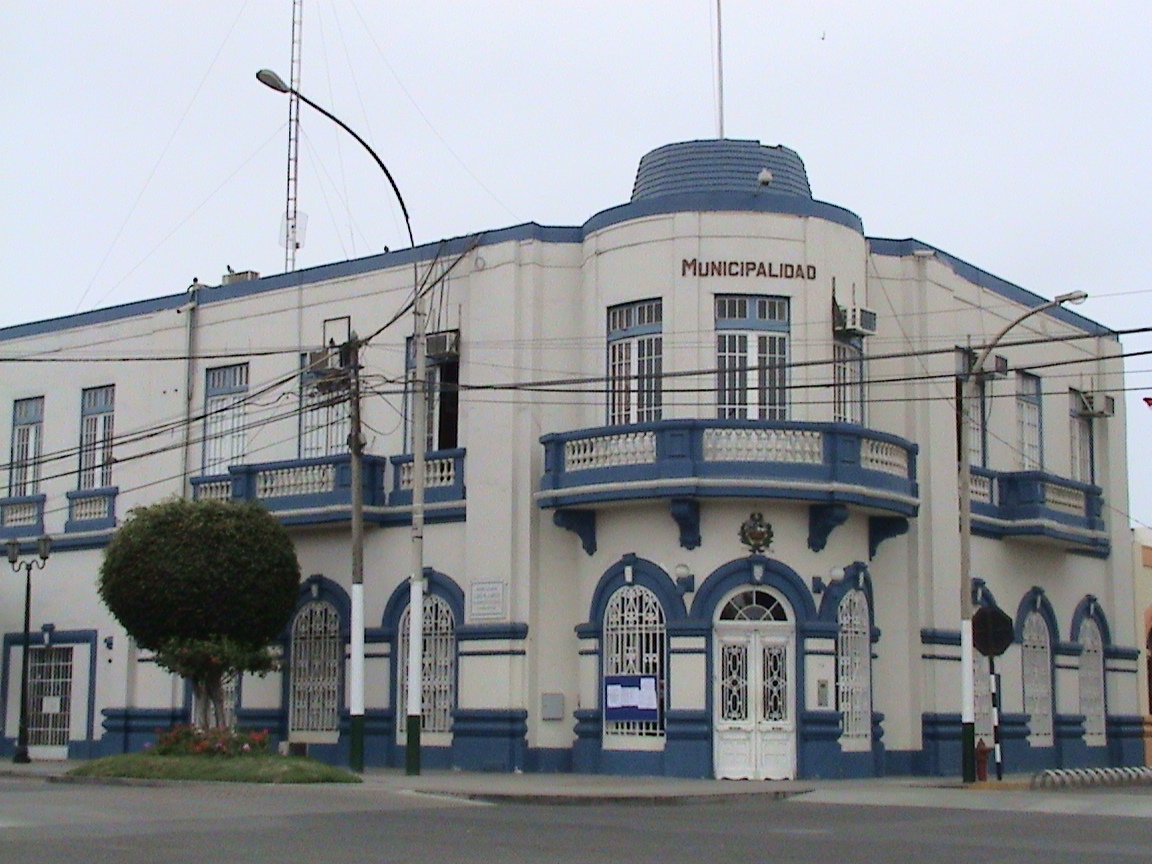The image captures an imposing, mostly white building set prominently on the corner of intersecting streets. Its architectural details include striking blue accents around the windows, doors, and balconies, with blue also adorning the roof. The main entrance, situated precisely at the corner, is flanked by tall windows protected with gate-like grilles reminiscent of jail cells. The second floor features balconies with white, decorative poles and the same blue trim. Prominently displayed on this floor is the word "Municipalidad" in maroon letters, indicating a municipal building, likely in a Spanish-speaking country. In front of the building, a neatly pruned tree in a ball shape and accompanying shrubs with small flowers add a touch of greenery to the otherwise architectural scene. Ornamental lampposts, a road sign on a black and white pole, and power lines crisscrossing above contribute to the urban setting. The street is notably devoid of cars, showcasing a grey cement surface. Two towers or antennas are visible atop or behind the building, adding to the detailed complexity of the scene. The photograph appears to be taken from across the street, providing a comprehensive view of this corner edifice.